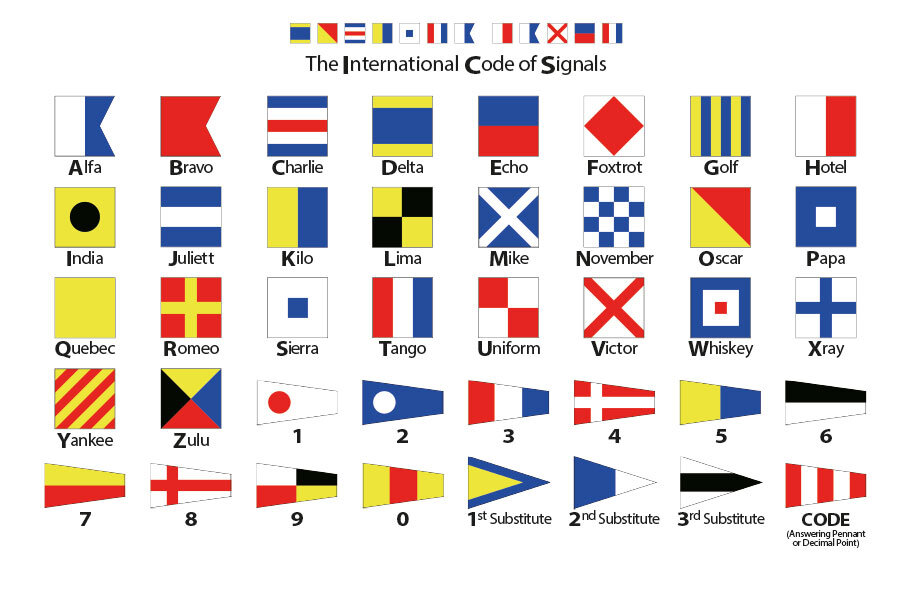The image prominently displays the International Code of Signals, with the title "International Code of Signals" written in black letters at the top. Below the title, there are multiple rows of signal flags, each representing a different letter from the nautical alphabet: Alpha, Bravo, Charlie, Delta, Echo, Foxtrot, Golf, Hotel, India, Juliet, Kilo, Lima, Mike, November, Oscar, Papa, Quebec, Romeo, Sierra, Tango, Uniform, Victor, Whiskey, X-Ray, Yankee, and Zulu. Each flag is depicted in its distinct color pattern, such as Charlie having a blue, white, red, white, blue stripe pattern, and Delta with a yellow, blue, yellow pattern. Additionally, numerical flags and symbols are included, illustrating the full scope of how these signals are used in maritime communication. The image serves as a detailed visual guide to the various flags and their corresponding meanings in the International Code of Signals.